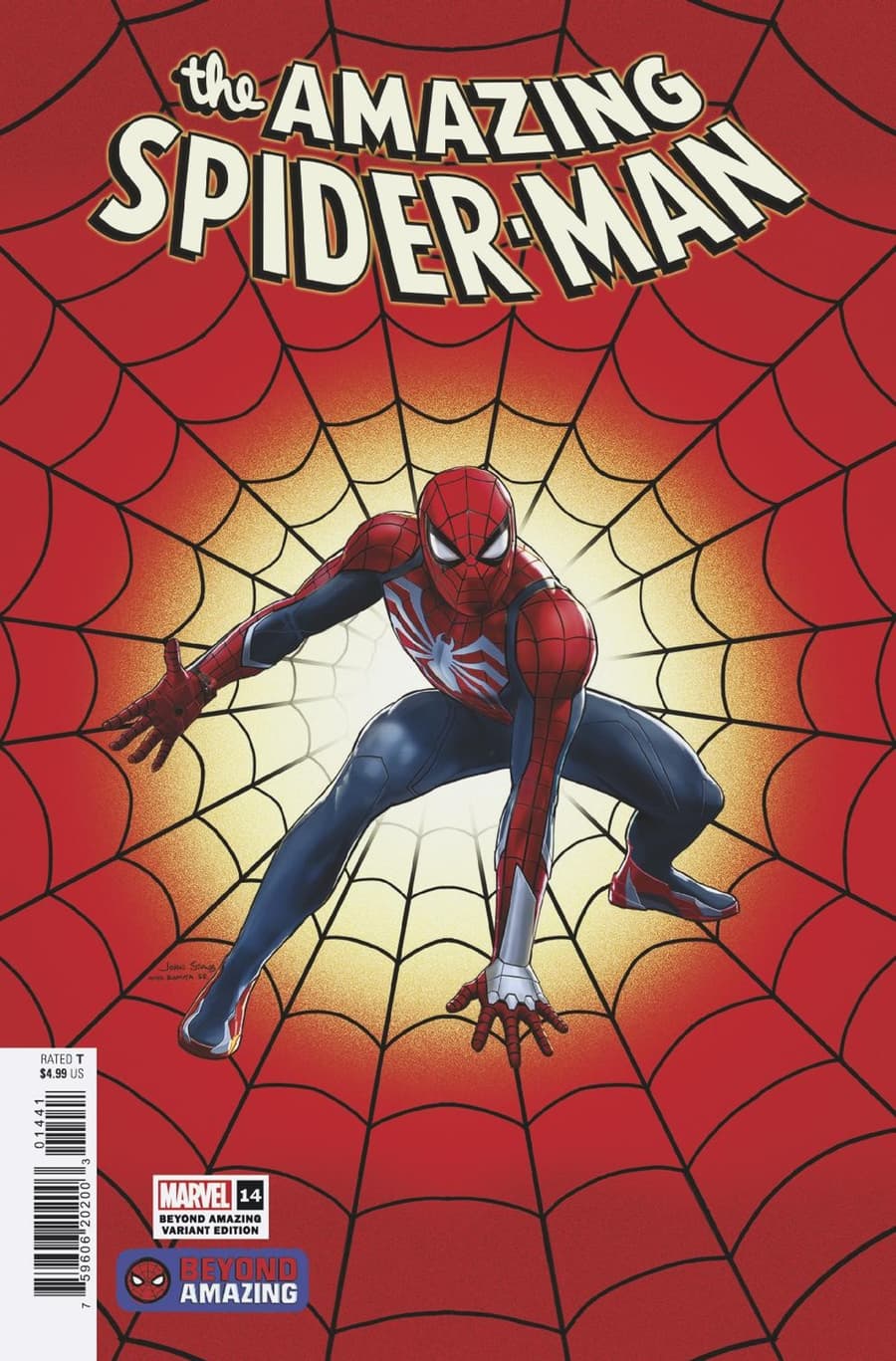This detailed cover art of the comic book titled "The Amazing Spider-Man" is striking and visually engaging. The background is predominantly red with a radiant yellow glow emanating from the center, enveloped by a black spiderweb design that forms a circle around it. At the heart of this circular design, Spider-Man is depicted in a dynamic crouching stance, ready to spring into action. His left arm is extended forward, touching the ground, while his right arm is positioned behind him, poised as if about to shoot webbing. Spider-Man’s costume features blue tight pants and a red shirt adorned with intricate black web patterns, complemented by blue stripes on the sleeves. His mask matches his suit, showcasing white eyes outlined in black with sharp points at the top, and his chest bears a prominent white stylized spider symbol.

The top of the cover is adorned with the title "The Amazing Spider-Man" in curved yellow text with a black shadow, enhancing its visibility against the red background. In the bottom left corner, several labels are present: a vertical white rectangle indicating "Rated T for $4.99 US" accompanied by two barcodes. Adjacent to these, there is a white horizontal box containing a red box with "Marvel" in white text, a black box with "14" in white text, and the inscription "Beyond Amazing Variant Edition" in black text. Additionally, a rounded bluish-purple box displays an icon of Spider-Man on the left, with the words "Beyond" in red text and "Amazing" in white text beneath it. This meticulously designed cover not only captures the essence of Spider-Man but also intrigues the viewer with its vibrant and detailed artistry.